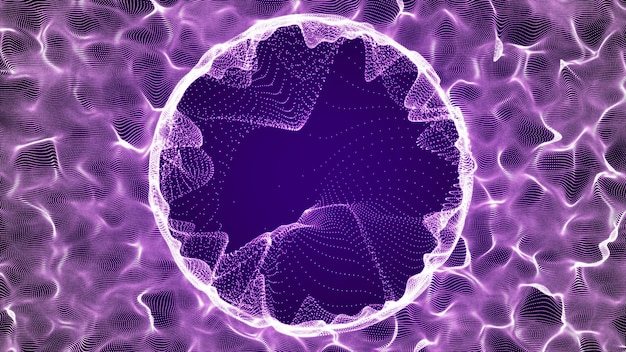The image is a computer-generated, abstract rectangular artwork, measuring approximately 3.5 inches by 5 inches. Dominating the center of the image is a large, ghostly white circle that appears to fade in and out, creating a translucent effect. Within this circle, there is a bluish-purple hue. Surrounding and extending beyond the circle are repetitive, deep purple shapes resembling sound waves or wavelength designs, which are accentuated with white and black shadowing. These shapes create a netting or tunnel-like appearance, giving the image a dynamic and layered look. The overall style feels like a visual representation of sound waves, with the central circle and the surrounding patterns harmonizing in varying shades of purple and violet. Despite its repetitive nature, the image's combination of colors and shapes provides a captivating abstract visual experience.